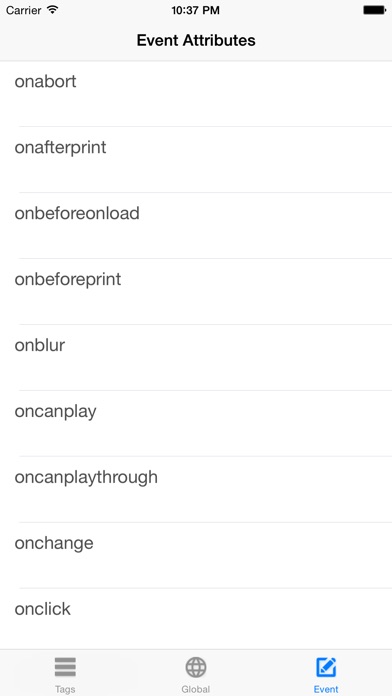The image is a screenshot captured on a smartphone, showcasing a specific application interface. The screenshot reveals a full Wi-Fi connection, indicated by the signal bars in the top right corner next to the carrier's name. To the left of the Wi-Fi icon, the time is displayed as 10:36 PM. The battery icon, positioned to the far right, indicates a fully charged battery.

The main focus of the screenshot is a page titled "Event Attributes." This section lists various event triggers written in black text, each separated by a dividing line. The events listed include:

- onAbort
- onAfterPrint
- onBeforeUnload
- onBeforePrint
- onBlur
- onCanPlay
- onCanPlayThrough
- onChange
- onClick

At the bottom of the screen, there are three navigation options: "Tags," represented by an icon of three stacked lines, "Global," represented by an earth icon, and "Event," where the current page is being shown, indicated by blue text and a blue square icon with a pencil. The background color of the entire page is white, providing a clean and clear viewing experience.